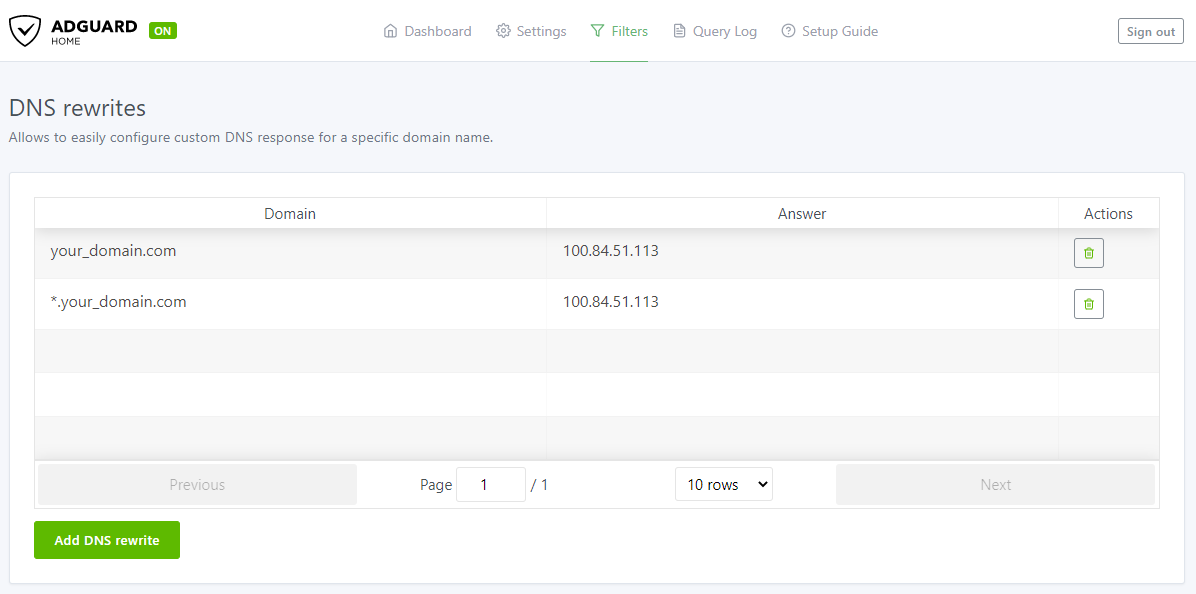The image depicts a web page titled "AdGuard Home" prominently featuring the AdGuard logo on the top left—a shield with a black checkmark inside. Adjacent to the logo, the text "AdGuard Home" is displayed, accompanied by a green indicator labeled "On." The top navigation menu includes options for "Dashboard," "Settings," "Filters," "Query Log," "Setup Guide," and a "Sign Out" button positioned at the top right corner.

In the main content area under the heading "DNS Rewrites," a brief description explains that this feature allows users to easily configure custom DNS responses for specific domain names. Below this description is a structured chart with the columns labeled "Domain," "Answer," and "Actions."

The first entry in the chart lists "Your_Domain.com" under "Domain" with the IP address "100.84.51.113" under "Answer." The "Actions" column contains an icon of a trash can. The second entry follows a similar structure with "Asterisk.Your_Domain.com" under "Domain" and the same IP address "100.84.51.113" under "Answer," also accompanied by a trash can icon in the "Actions" column.

At the bottom of the chart, pagination details indicate "Page 1 of 1," showing 10 rows per page. Finally, a green button with white text at the bottom left corner reads "Add DNS Rewrite."